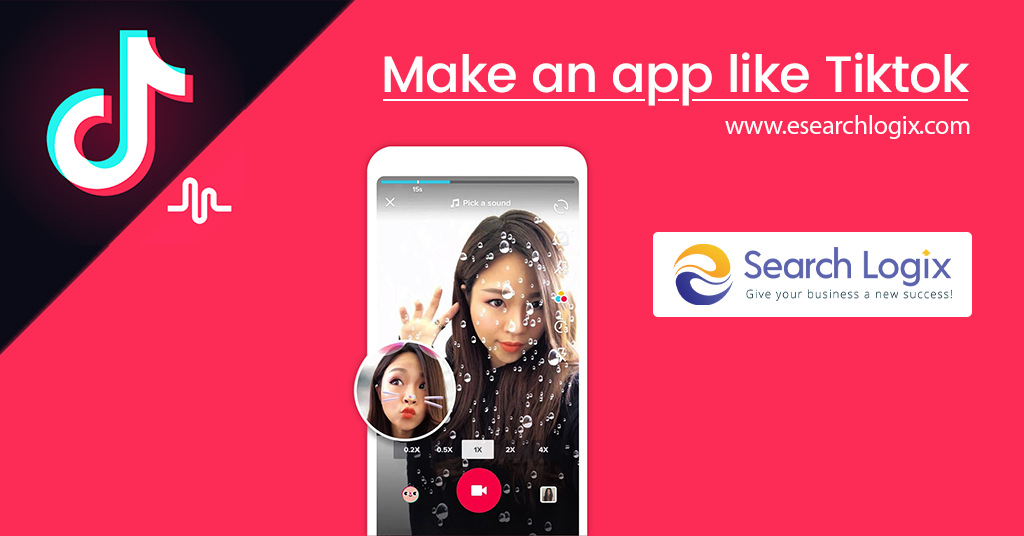### Caption:

This image is an advertisement for creating an app similar to TikTok. The upper left-hand corner features the TikTok logo, a lowercase cursive "t" outlined in blue and red with a white center, set against a black background. The rest of the image's background is red. To the right of the TikTok logo is a white squiggly line resembling a pulse wave. At the top of the red background, bold white text reads, "Make an app like TikTok," with "Make" and "TikTok" starting with capital letters and underlined in white.

Below the text is a website address: "www.searchlogics.com". Beneath the address is an image of a smartphone displaying what appears to be a TikTok video interface. The phone's screen has a gray background with a blue progress bar indicating 15 seconds. On the left side is an "X", and in the middle is a musical note icon with the text "Pick a sound," flanked by two circular arrows. A brunette Asian female is featured on the screen, posed with her right hand by her head, wearing a black sweater and red lipstick. She has a raindrop filter applied to her image.

In the far right of the phone screen, various icons are almost visible, including a magnifying glass and circles in yellow, red, and blue, alongside a clock. Overlaid on the bottom part of the phone image, the same woman is shown making a duck face with a filter adding whiskers and a nose, looking off to the side.

At the bottom of the phone screen, speed options appear (0.2x, 0.5x, 1x, 2x, 4x), with the "1x" option highlighted in gray. The bottom left corner features a circle with an animal face, showing eyes and a beak. In the center is a red recording button with a white camera icon. Next to it is a square preview of saved images on the phone. To the right of the recording button is a white bar with a red-gold and red-purple circular formation displaying the company name "Search Logix" with a gold diamond over the "i". Below that, it says, "Give your business a new success."